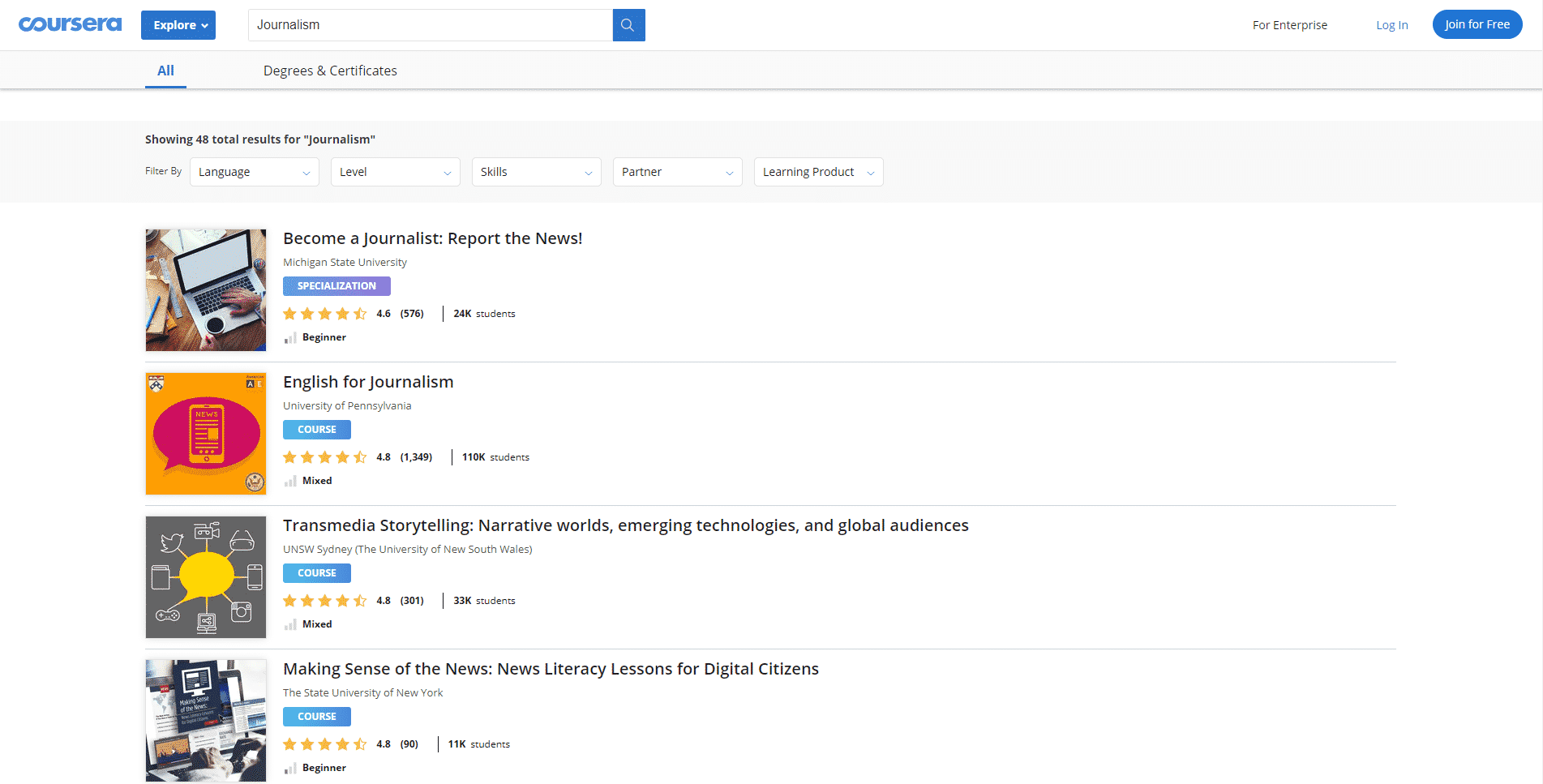In the top left corner of the image, a blue emblem reads "Coursera." Directly below, a blue button labeled "Explore" is present, beside a search box with the placeholder text "Journalism." Beneath the search box, options labeled "All," "Degrees and Certificates" are displayed. Further down, the text "Showing 48 Total Results for Journalism" is visible. Below this, there are filter options for "Language," "Level," "Skills," "Partner," and "Learning Product," each encapsulated within a box featuring a drop-down menu.

The main section of the image features thumbnails on the left, showcasing four distinct courses. The descriptions for each course are as follows, from top to bottom:

1. "Become a Journalist: Report the News" by Michigan State University. This specialization course boasts a rating of 4.5 stars, gathered from 579 reviews, and has enrolled 34,000 students. It is categorized at the beginner level.

2. "English for Journalism" offered by the University of Pennsylvania. This course has a rating of 4.3 stars based on 1,349 reviews and serves 110,000 students.

Each course listing includes a detailed thumbnail on the left side.